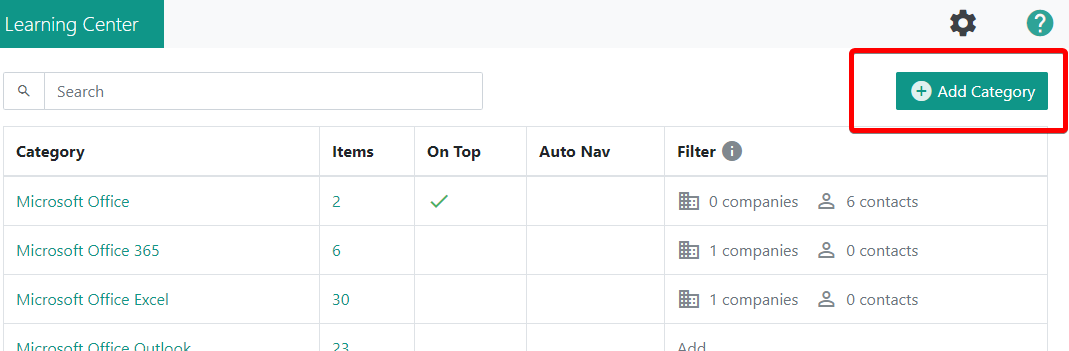The screenshot depicts a webpage from the "Learning Center" with a greenish-blue banner at the top displaying the text "Learning Center" in white. On the right-hand side of the banner, there is a black gear icon followed by a white question mark encased in a circle, also in greenish-blue. Below the banner, on the left-hand side, is a search magnifying glass icon next to a white search box with the word "search" inside it.

Directly beneath the search box, there are several rows and columns with the column titles: "Category," "Items," "Auto Nav," and "Filter." The "Filter" column title has a grey circle with the letter 'I' in white, indicating that it provides more information upon hovering. These column titles are in black text.

Listed under the "Category" column, the text is greenish-blue and includes:
- Microsoft Office
- Microsoft Office 365
- Microsoft Office Excel
- Microsoft Office Outlook

Next to these categories in the "Items" column, corresponding numbers in greenish-blue read:
- 2
- 6
- 30
- 23

The first entry under "Category" (Microsoft Office) has a greenish-blue checkmark, indicating selection. The "Auto Nav" column is visibly empty. The webpage is designed to be interactive, likely aimed at helping users navigate through various learning resources related to Microsoft Office products.